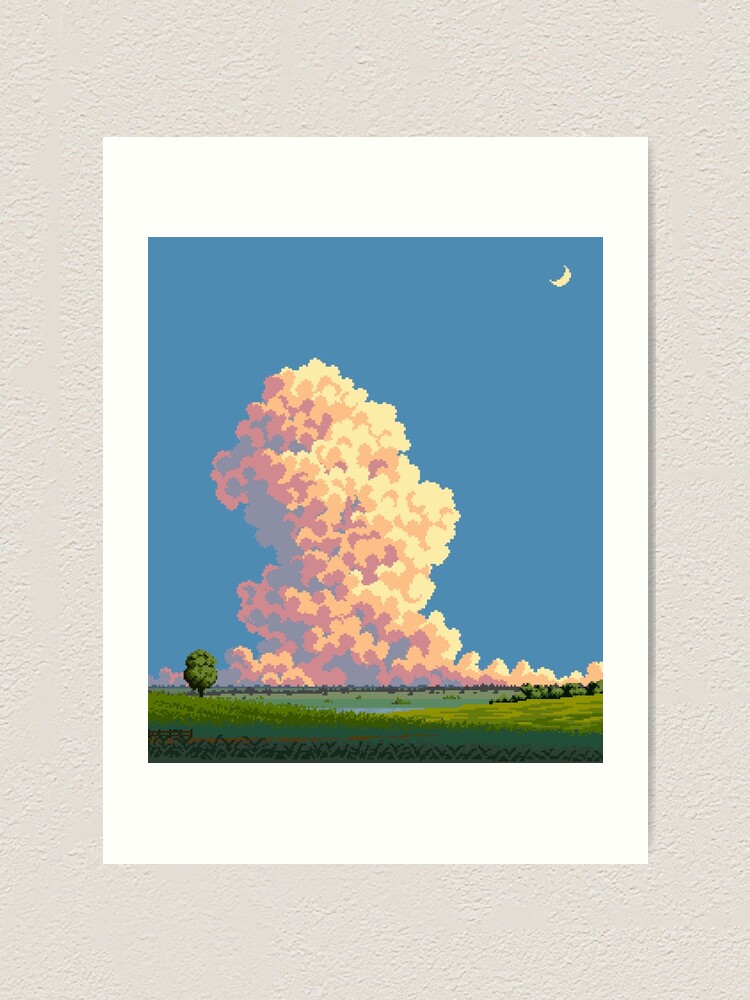A painting is displayed on a textured, stucco-like wall of a darker off-white color. The painting is set against a white background, resembling a poster. In the center of the composition, a rectangular piece of pixel art captures attention. The scene within the painting unfolds under a deep blue sky, punctuated by a yellow crescent moon in the top right corner. Dominating the center is a towering cloud formation with color gradients from light lavender on the left, transitioning through orange and reddish highlights, to a pale yellow on the right. The cloud's texture evokes an abstract yet detailed appearance, adding to the scene's dramatic effect. Below, a rolling green field stretches across the bottom, varying in shades with darker greens at the base and lighter hues upwards and to the right. A solitary green tree stands prominently on the left, while a small scattering of trees dots the distant horizon, enhancing the serene landscape.